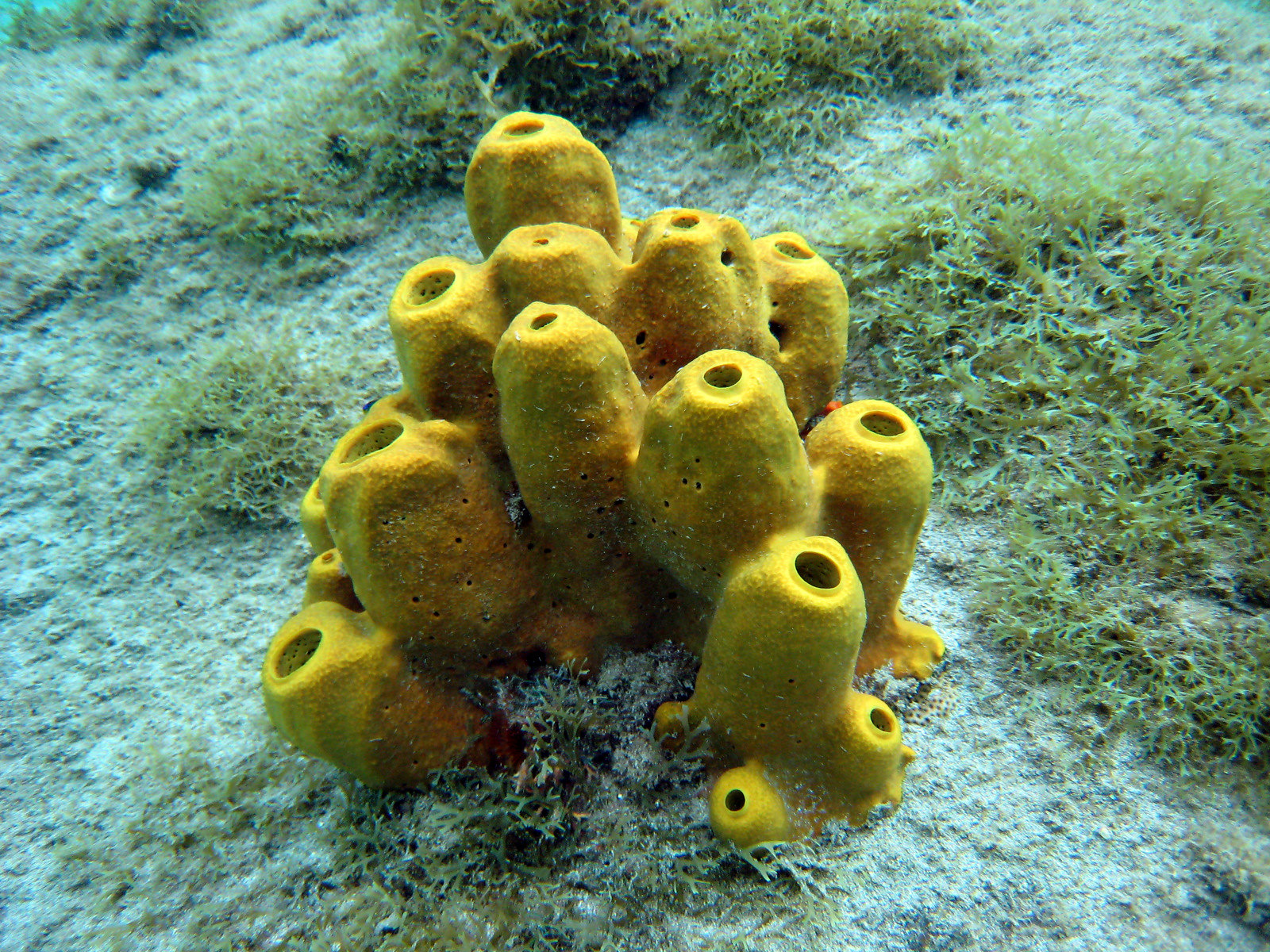The underwater scene showcases a vibrant collection of cylindrical yellow coral structures resembling man-made objects with near-perfect central holes and smaller drilled-like side openings. These clusters of coral, intriguingly bright yellow, are densely packed, with the taller tubes in the center and shorter ones on the periphery, forming a striking focal point in the high-quality image. The coral rests on a patchy ocean floor featuring a mix of green algae, seaweed, and lighter brown sandy areas. Surrounding the vibrant yellow coral are patches of white coral, suggesting possible bleaching among the natural reef formations. This detailed portrayal captures the essence of an intriguing and possibly artificial feature on the seabed, blending with the natural marine ecosystem.